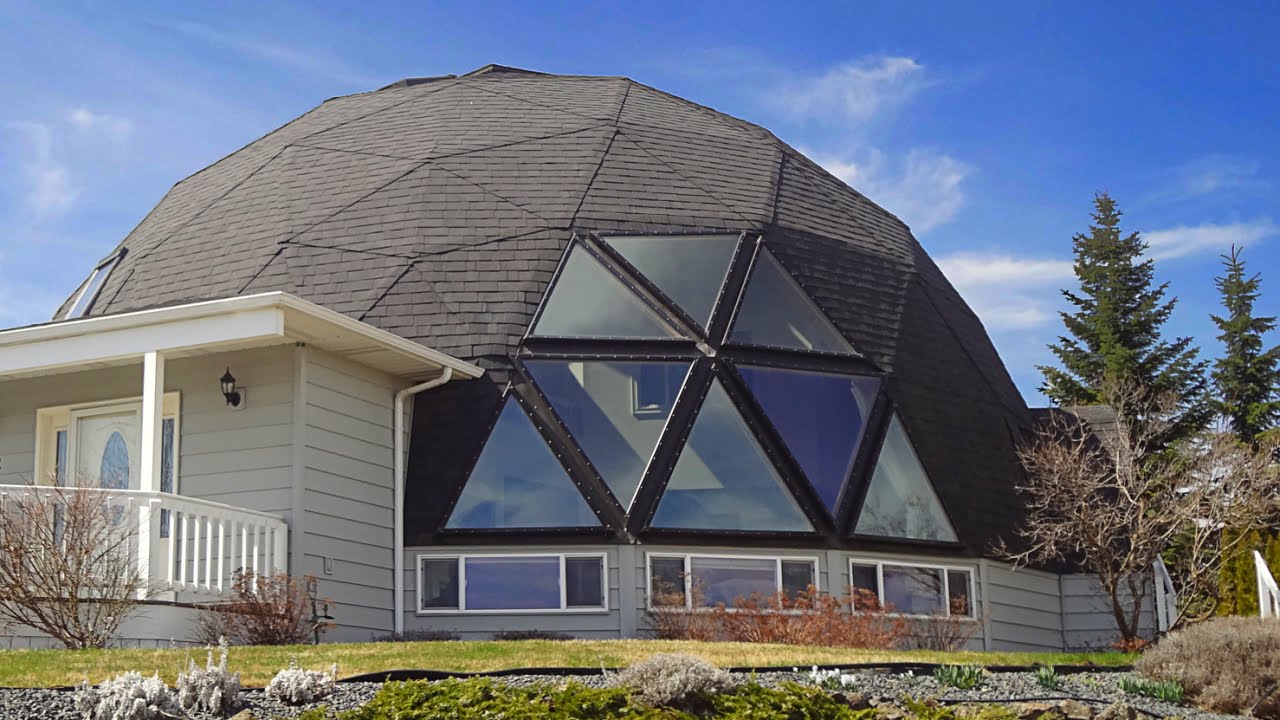This photograph captures a uniquely styled house, combining traditional and modern architectural elements against a backdrop of clear blue skies. The front of the house features a typical design with a pale beige exterior, a white-trimmed front door, and a wraparound porch with white railings. This conventional facade stands in stark contrast to the house's right side, where a striking, black dome-shaped structure emerges. This dome is constructed from geometric shapes, predominantly triangles, and squares, with many of the triangles made of glass. The glass triangles are framed in black and oriented in various directions, creating an intricate pattern. Below the dome, there are several rectangular glass windows framed by shutters, which give the appearance of a regular bottom floor or basement. The scene is complemented by two tall green trees on the right side of the house, adding a natural element to the innovative design. The ground is a mix of gravel and grass with small plants, providing a simplistic yet charming foreground.